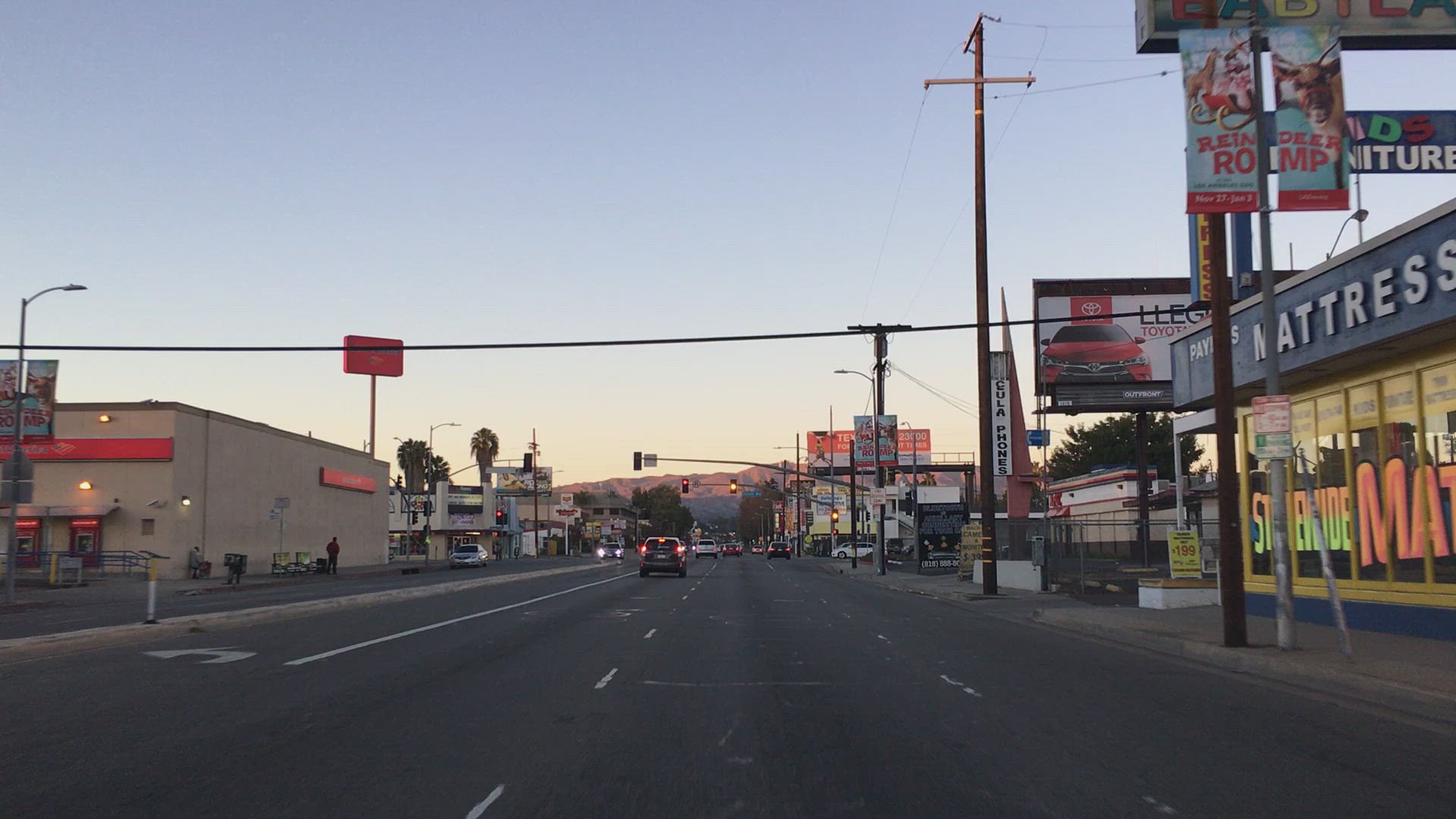The photograph captures a bustling city street at sunset, casting a slightly smoggy blue sky transitioning to light blue and faint orange hues. The street, which recedes into the distance, is a multi-lane roadway featuring two lanes on this side, a left turning lane, and a potential safety lane. Centered in the image is a car with its brake lights on, stopped under a red traffic light at an intersection. Surrounding the road are various commercial buildings, including a prominently visible mattress store with glass windows and a painted sign that partially reads "MAT." To the right, commercial establishments line the street, while on the left, a large beige building with red trim and signage exists. Several street elements are present, such as telephone poles with lights, billboards, street signs, and banners promoting a "Reindeer Romp" event. Tall trees intermingle with the buildings, adding greenery to the scene. Above the street, a wire stretches between poles, disappearing off to the left of the image. In the distance, the backdrop features a mountain range with brown peaks subtly illuminated by the fading sunlight. The overall scene conveys a transitioning time of day in a vibrant urban setting.